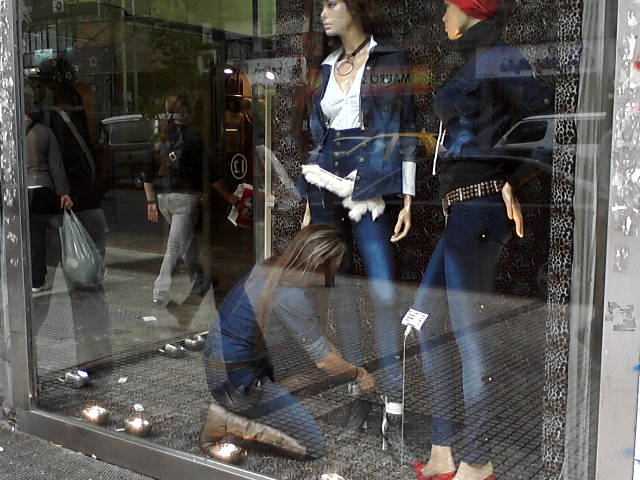This detailed color photograph, captured in landscape orientation, shows a storefront display of a clothing shop viewed from the sidewalk. The image is filled with reflections that reveal cars and pedestrians on the opposite side of the street, adding depth to the scene. Inside the dark gray window frame, which is adorned with a leopard print inner border, a girl with long dark hair accented with gold streaks is kneeling and working attentively on two mannequins. She is dressed in a gray roll-up sleeve shirt, blue jeans, and beige boots. The mannequins, situated on the right side, are both styled in coordinated blue denim jackets and pants. The mannequin on the left is paired with a white shirt and a bold silver necklace, while the one on the right, facing the other mannequin, sports a red cap. The window dresser is focused intently on adjusting the clothing at the mannequin's foot, contributing to the realistic and representational nature of the scene.